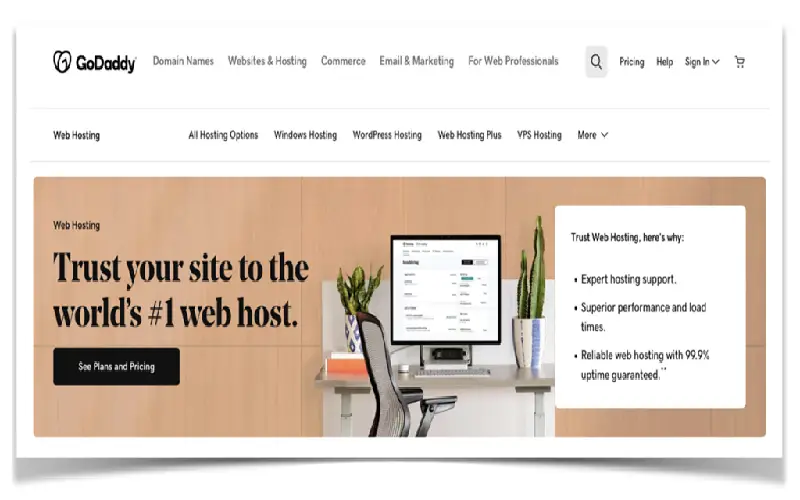This is a detailed, cleaned-up caption for the described web image:

---

The image features a clean white background with subtle gray shadows cast under the bottom left and right corners. At the top left, the GoDaddy logo is prominently displayed, accompanied by the text "GoDaddy." Adjacent to the logo in a horizontal line, the categories "Domain Names," "Websites & Hosting," "Commerce," "Email & Marketing," and "For Web Professionals" are listed. Further along this header, a highlighted search icon is visible, followed by the options "Pricing," "Help," and "Sign In," the latter featuring a drop-down arrow. A shopping cart icon concludes this section.

Below this main header, a smaller secondary header spans the width of the image. It includes navigation items from left to right: "Web Hosting," "All Hosting Options," "Windows Hosting," "WordPress Hosting," "Web Hosting Plus," "VPS Hosting," and a "More" button.

The bottom section of the image showcases an illustration of a workspace, featuring a laptop or desktop computer, a keyboard, and a table with a chair flanked by two potted plants. To the left of this illustration, bold black text declares, "Trust Your Site to the World's Number One Web Host." Directly beneath this, a black horizontal button reads "See Plans and Pricing."

On the right side of the image, a pop-up white box provides compelling reasons to choose GoDaddy's web hosting services. It highlights "Expert Hosting Support," "Superior Performance and Load Times," and "Reliable Web Hosting with 99.9% Uptime Guaranteed." The background behind the illustration of the workspace is a warm, light brownish orange hue.

---